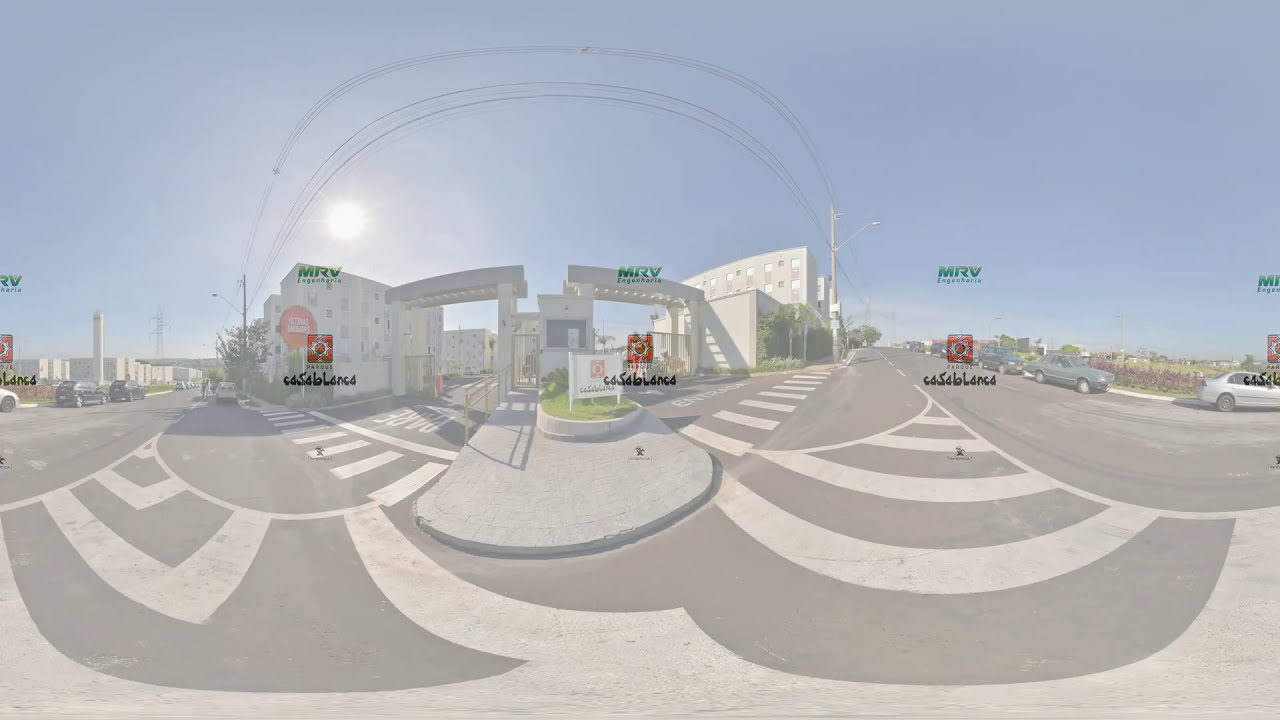The image displays a light gray asphalt road with clearly marked white crosswalks, captured in a panoramic, convex style that curves the roads, skies, and buildings. On the right side of the street, several cars—a white car, a darker gray car, and a blue car—are driving. The scene is bathed in sunlight from a clear blue sky, with the sun positioned on the left. Dominating the background are white buildings adorned with windows; one of these buildings features framed archways leading into what appears to be a parking garage. In the middle, a circular berm sidewalk separates the dual lanes, facilitating multiple crosswalks. The foreground is devoid of people but includes street lights, power lines, and trees. There is text visible across the image: four identical green "MRV" labels, each above a red square containing a red circle, and below that, in black lettering, it says "Casablanca."